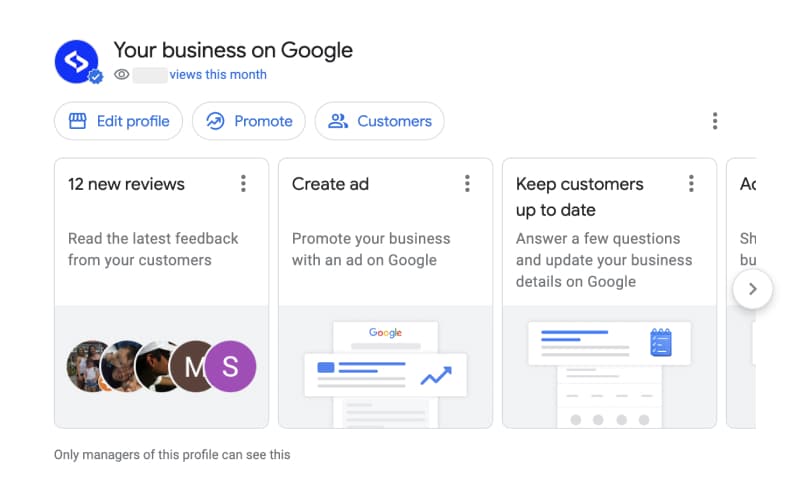This image displays various elements on a white background, organized primarily within a structured, user-interface layout related to managing a Google business profile.

In the upper left corner, there is a blue circle containing two sideways V's pointing towards each other, alongside a tiny circle with a check mark. The text "Your business on Google" is displayed in black next to this icon. Below this, there appears to be a small "CBS" logo in black and a gray box, followed by the phrase "Views this month" in blue.

The main layout includes several white boxes outlined in gray. The first box contains the blue text "Edit Profile," and features an additional smaller box. Another gray-outlined box with white inside and blue text reads "Promote" and includes a circle with a wiggly arrow. The next box, labeled "Customers," also has three black dots aligned vertically on the right side.

Beneath these, there are three larger rectangular sections with white tops and light blue bottoms. The first section announces "12 new reviews" and encourages viewing the latest feedback from customers. It includes five small circles, with three containing people's avatars and the last two marked with an "M" and an "S," the latter being purple with a white "S."

The second large section reads "Create ad" and invites users to promote their business with a Google ad. It includes three dots and an icon of a piece of paper with the Google insignia. Below this, a small blue box, two blue lines, and a blue arrow are illustrated.

The third section is titled "Keep customers up-to-date" and prompts users to answer questions and update business details on Google. There is an accompanying icon of a piece of paper with blue elements that resemble a calendar.

The lower part of the layout reveals another white area with a gray circle containing a white arrow pointing to the right. There is a partial view of an additional box. The text at the bottom of the image states: "Only managers of this profile can see this."